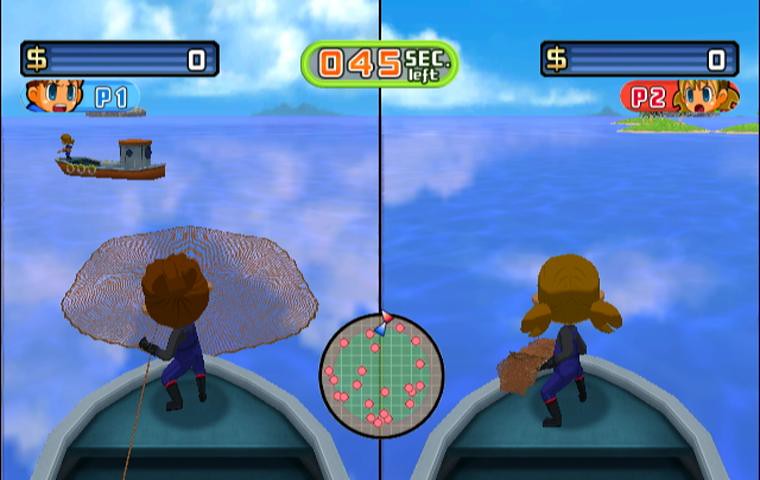This image is a split-screen snapshot from a video game featuring two players, one male and one female, standing back-to-back on the prow of a semi-circular, boat-like platform. The left screen identifies the boy as "Player 1" with an anime-style icon and the text "P1". The right screen labels the girl as "Player 2" with a corresponding icon and the text "P2". Both players are dressed in black jumpsuits with blue bodies and red stripes; the boy has short brown hair while the girl sports two brown pigtails. A map at the top center highlights each player's location with arrows and red dots. The scene is set in a misty, water-filled area with clouds, distant mountains, and some grassland near Player 2. Each screen has a box displaying "$0" in the top corners, and a countdown timer across the middle indicates "45 seconds left". The boy on the left is seen casting a net into the water, and the girl on the right appears to be retrieving something from it, engaging in what seems to be a cooperative or competitive task within this serene yet strategical environment.